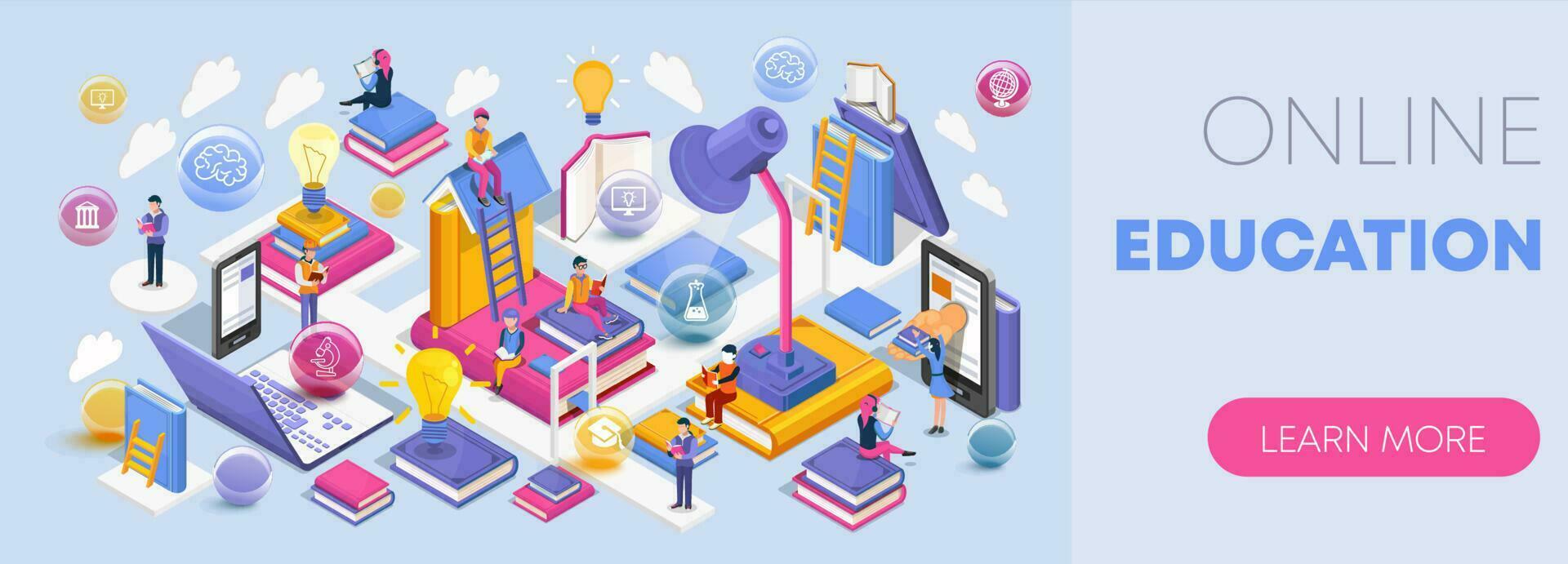The image is a professionally rendered ad for online education, featuring a vibrant and detailed graphical design. On the right-hand side, the text "ONLINE EDUCATION" is displayed, with "ONLINE" in black and "EDUCATION" in blue. Beneath this is a pink oval button with a white "LEARN MORE" inscription. The background is sky blue, and the main colors throughout the image include blue, pink, purple, yellow, and white.

The scene depicts various cartoon figures, approximately half a dozen, engaging in different educational activities. These characters are standing, sitting, and reading amidst an assortment of books, each adorned with light bulbs to symbolize the acquisition of ideas. One notable figure has climbed a ladder and is perched atop a small house, while another woman sits on a tall stack of books reading. 

There are additional graphical elements, such as laptops, ladders, lamps, clouds, and circles containing symbols like a globe, a brain, a building, and a telescope. A prominent light shines on the characters, emphasizing their learning environments. The image is professionally crafted and does not contain any other text indicating the company's name.